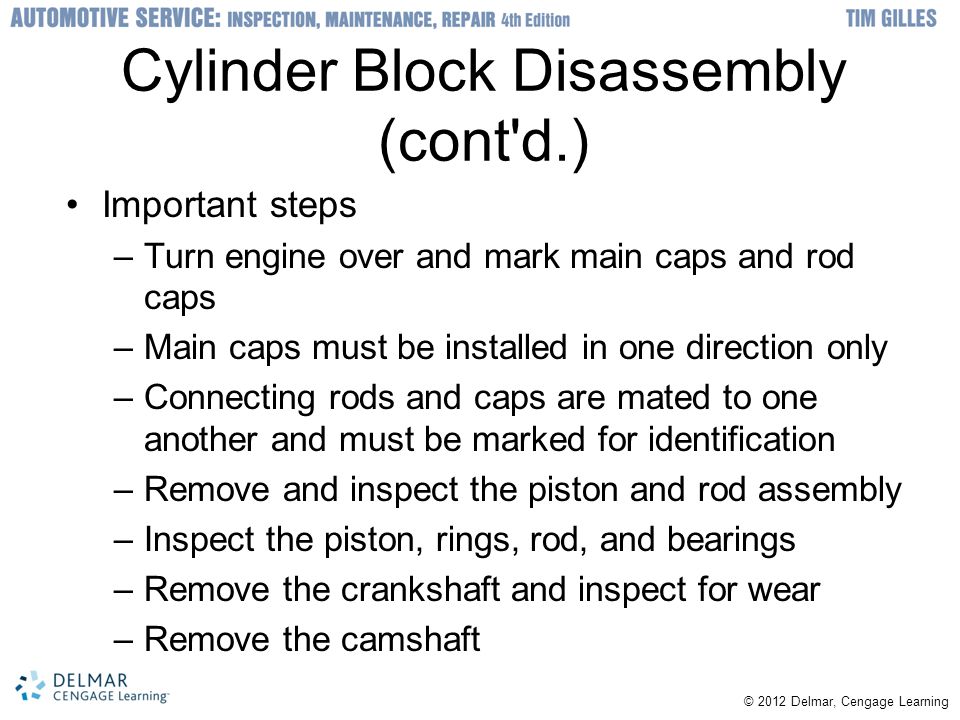The image presents a detailed instructional text from a manual or presentation slide on a white background. At the very top, in blue lettering, it reads, "Automotive Service: Inspection Maintenance Repair, 4th Edition, Tim Gilles." Below this, in larger black font, it states, "Cylinder Block Disassembly (Continued)." The section titled "Important Steps" follows with a bullet-point list of instructions: 
1. Turn engine over and mark main caps and rod caps.
2. Main caps must be installed in one direction only.
3. Connecting rods and caps are mated to one another and must be marked for identification.
4. Remove and inspect the piston and rod assembly.
5. Inspect the piston, rings, rods, and bearings.
6. Remove the crankshaft and inspect for wear.
7. Remove the camshaft.

The bottom right corner notes "Copyright 2012, Delmar Cengage Learning," while the lower left corner features the Delmar Cengage Learning logo, described as a spiral or circle of colored blocks accompanied by the company name in blue font. Overall, the image resembles a page from a technical manual or a slide from a presentation.